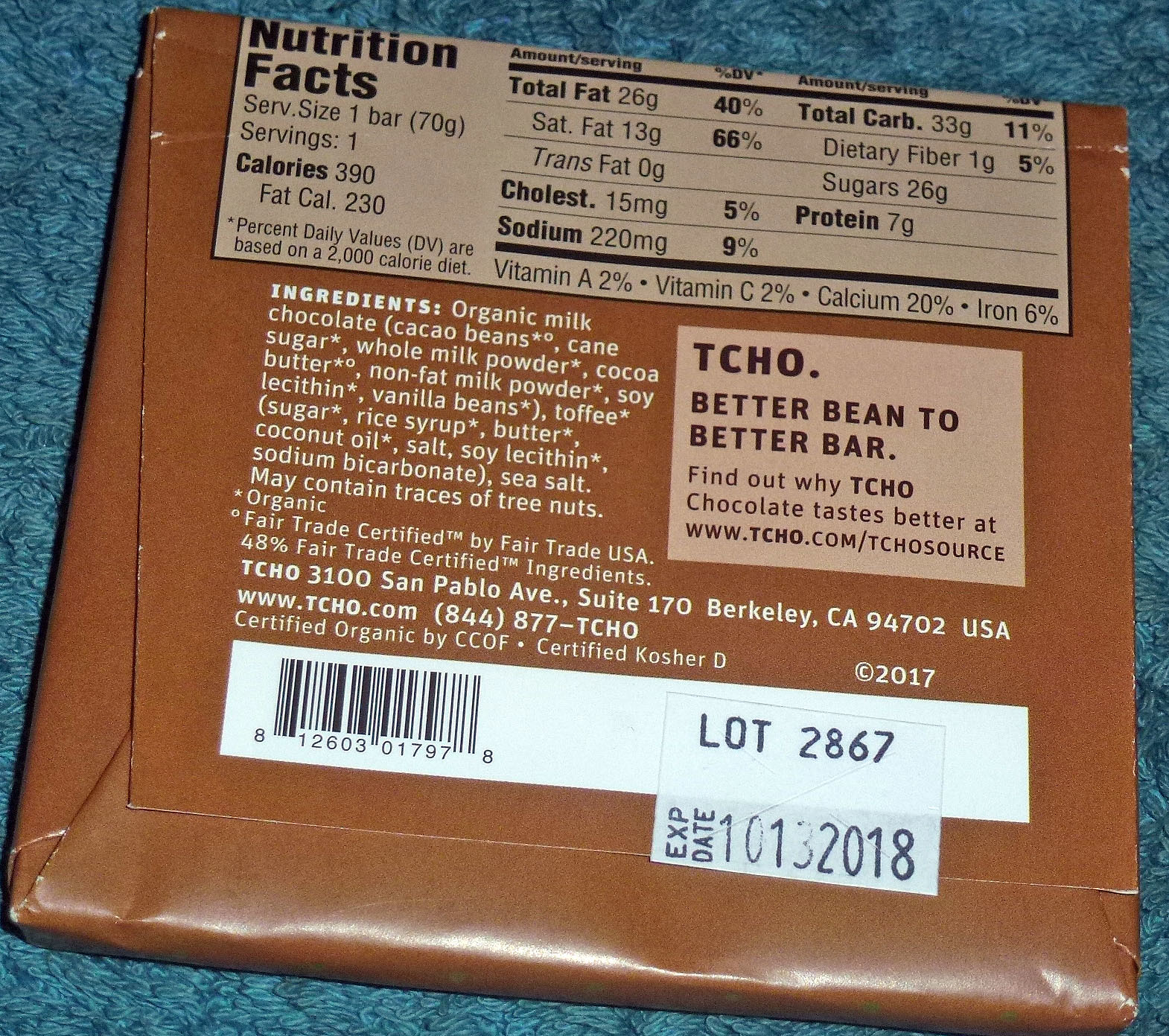The image depicts the back of a square candy bar, likely chocolate, in a brown paper wrapper. This wrapper, which seems to mimic the appearance of chocolate, lies on a blue and black splotchy surface, possibly a carpet or granite tabletop. The packaging features a lighter brown section at the top containing the nutrition facts in black text, listing details such as total fat, saturated fat, and cholesterol. Below this, the ingredients are printed in white text directly on the brown wrapper. To the mid-right section of the wrapper, there is a light brown square with black text that reads, "TCHO, better bean to better bar. Find out why TCHO chocolate tastes better at the TCHO website," suggesting the brand of the candy bar. Towards the bottom right corner, a white sticker displays the lot number "LOT 2867" and the expiration date "EXP date 10-13-2018." Additionally, a white barcode is seen on a white panel crossing the lower part of the wrapper. The overall setup of the image provides a detailed view focusing on the back side of the chocolate bar's packaging.